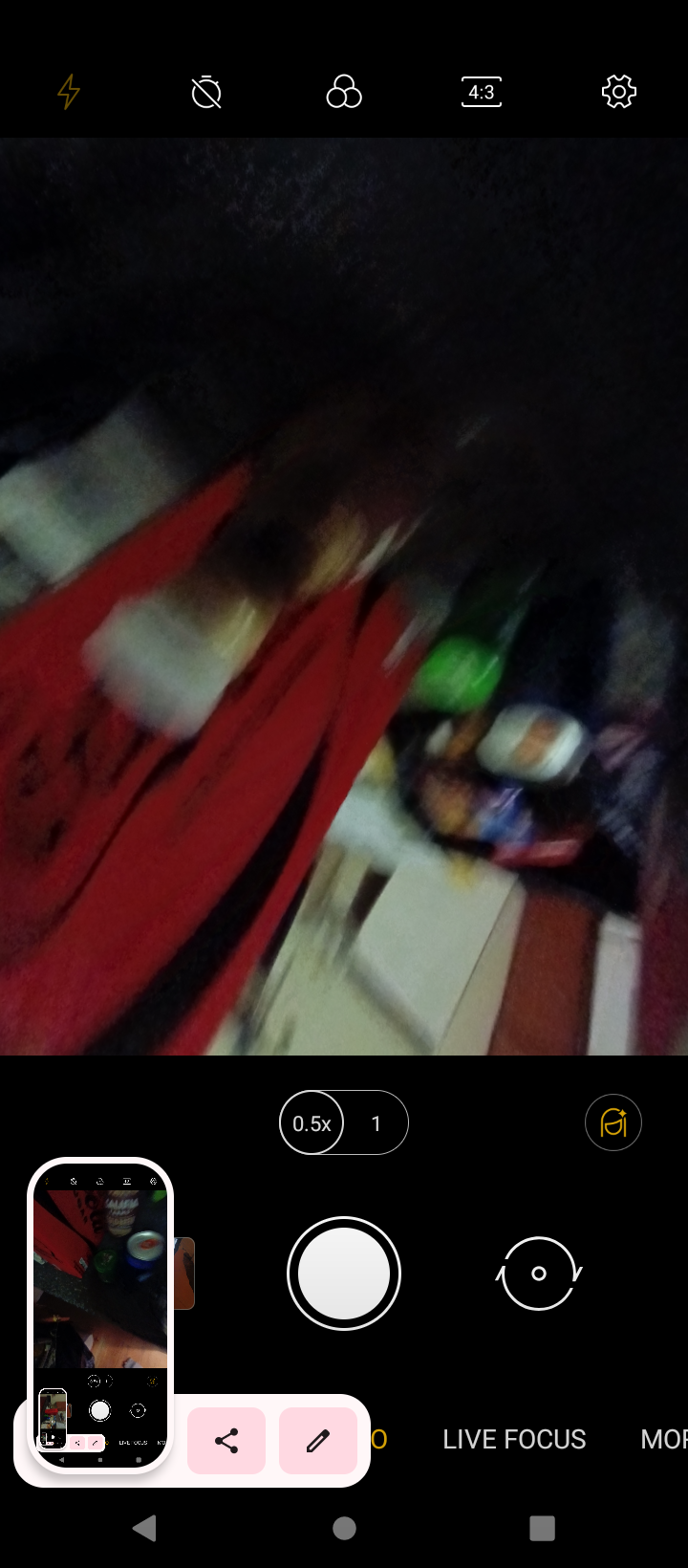This image depicts a blurry and out-of-focus screenshot taken within the camera app of an Android phone, indicated by the familiar navigation buttons—a triangle, a circle, and a square—at the bottom of the screen. The captured scene shows a cluttered room with various indistinct objects. At the very top of the screenshot are five icons related to camera settings: flash, timer, color balance, aspect ratio, and a gear icon for additional settings. The top third of the image appears predominantly black, and below that, there is a red dress with a black stripe, although it’s not in sharp focus. Scattered around the dress, there are what seem to be piles of paper, and further to the right, black luggage can be seen resting on a wooden floor. Additionally, at the bottom of the screenshot are the camera app’s interface elements, including an oval icon labeled "0.5," a "1" to its right, a large white shutter button, and a circular arrow icon for switching modes next to a smaller circle. In the bottom left corner of the screen, there's a small snapshot image of the photograph within the phone’s gallery, accompanied by a white bar containing share and edit buttons. The overall scene is chaotic and hard to interpret due to the motion blur and overlapping elements, with various potentially identifiable items such as jars, a ball of string, and other indistinct objects scattered throughout.